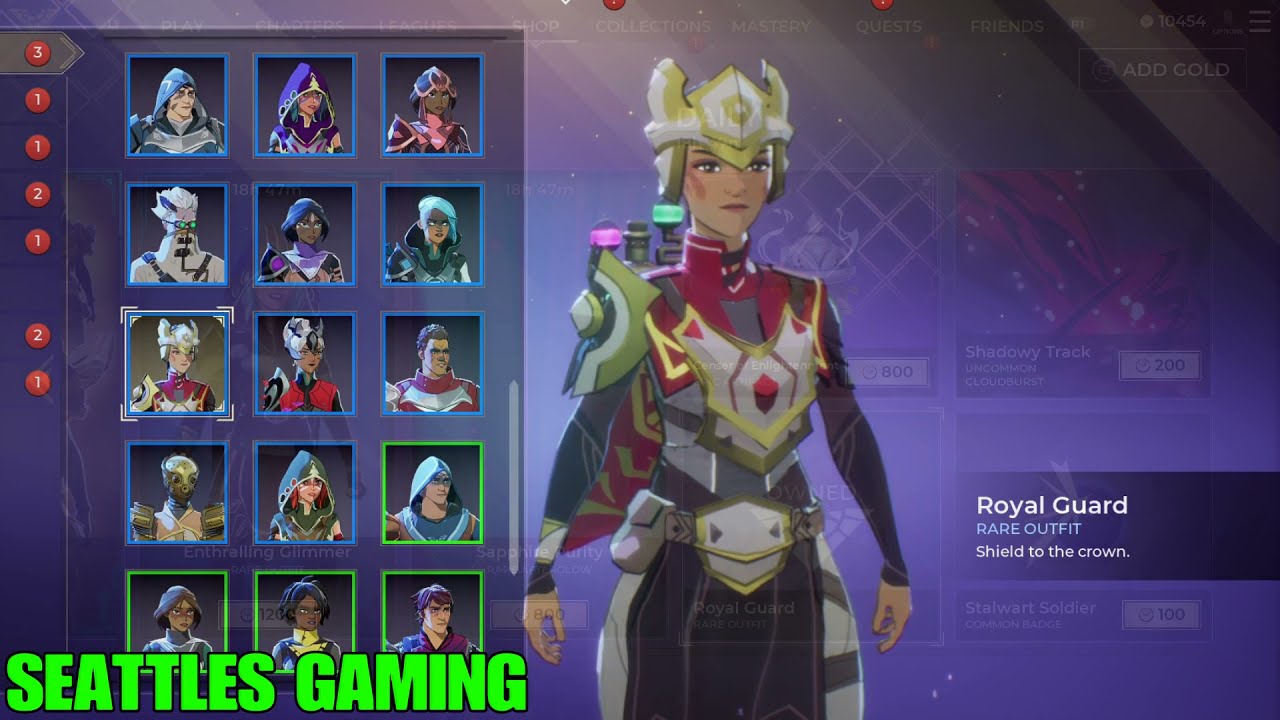The image is a detailed screenshot from a role-playing video game, depicting a character selection menu. The interface has a rich purple background. Dominating the center is a female character named the Royal Guard, distinguished by her opulent attire. She dons a white and yellow helmet resembling a crown, coupled with matching armor featuring intricate patterns and a red cape. Her ensemble includes a white and yellow chest piece, a belt with a central seal, and a shoulder pad on her right arm. Purple and green lights adorn her back, enhancing her regal appearance. On the left side of the screen, there are 15 smaller images of different characters available for selection. Key texts are present in bold green font; “Seattle's Gaming” is noted at the bottom right of the image, while on the right side, it reads, "Royal Guard wear an outfit sealed to the crown" emphasizing her prestigious status.